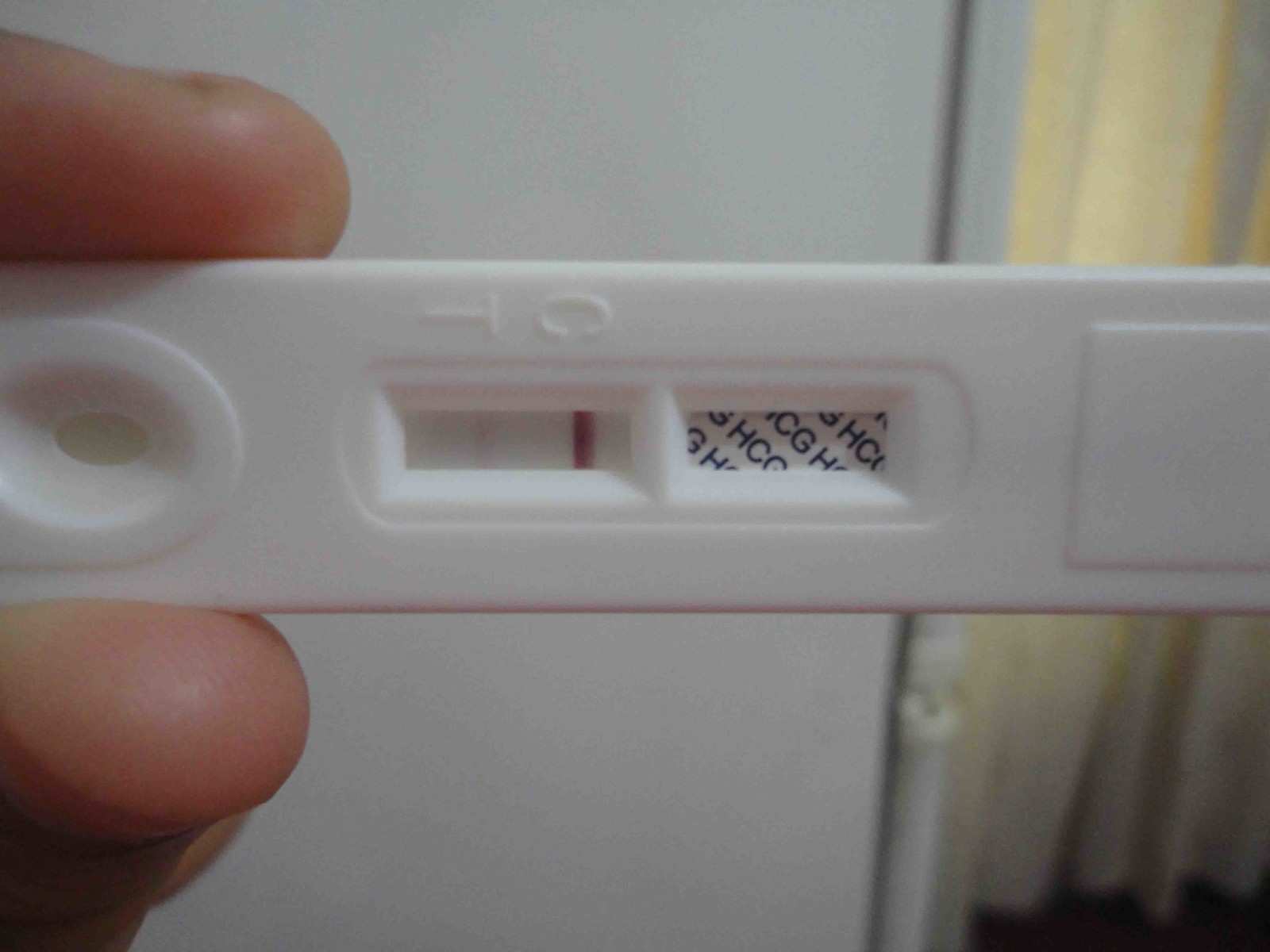A person is holding a diagnostic test in their hand, possibly a COVID-19 or HCG test. The image is in landscape orientation and appears to be a rectangle. The background features a wall, and in the upper right-hand corner, there is a yellow curtain with light filtering through it. The individual's hand, which has very short fingernails and light skin, occupies the foreground, holding the test device. The test device has a circular section between the fingers and two result windows. The first window displays one faint red line and one dark red line, situated below the letters "T" and "C", suggesting the possible interpretation of a positive "C" result. The second window is labeled "HCG". The image extends towards the right side, but the continuation of the test device fades from view.